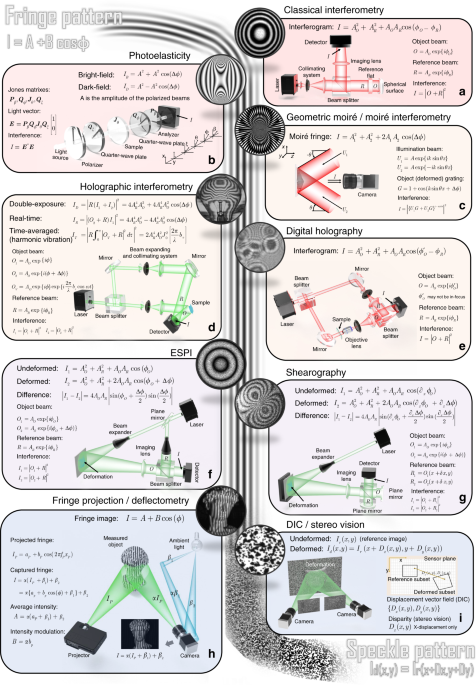The diagram showcases educational material focused on the concept of a fringe pattern, emphasizing the equation I = A + B cos θ. In the center, there is a black-and-white strip simulating a pipe through which dust particles move, depicted in nine individual circles with varying patterns in white, black, and gray. Surrounding this central strip are two columns of rectangular cells with rounded edges, each containing figures, equations, and text, although much of the text is blurred and difficult to read.

On the left side:
1. **Figure B**: A light pink box titled "Photoelasticity" with equations and figures.
2. **Figure D**: A light pink rectangular box titled "Holographic Interferometry" featuring figures in green and equations.
3. **Figure F**: A light gray box titled "ESPI," showing green-colored figures and equations.
4. **Figure H**: A blue-colored box labeled "Fringe Projection or Deflectometry," containing figures in green, blue, gray, and black, along with equations.

On the right side:
1. **Figure A**: A pink-colored box titled "Classical Interferometry" that includes figures and equations.
2. **Figure C**: A light pink box titled "Geometric Moiré Interferometry" with patterns in red and equations.
3. **Figure E**: A light pink box titled "Digital Holography" showcasing figures in red patterns and equations.
4. **Figure G**: A light gray box titled "Shearography," featuring green-colored figures and equations.
5. **Figure I**: A blue box titled "DIC/Stereo Vision," containing green and gray figures, equations, and a depiction of two cameras targeting a screen with green waves.

At the bottom right corner, a watermark reads "speckle pattern LD(X,Y) with respect to LR(X + DX,Y + DY)." The image combines mathematical inference, scientific visualization, and various interferometry methods, representing a detailed educational tool likely from a scientific textbook.